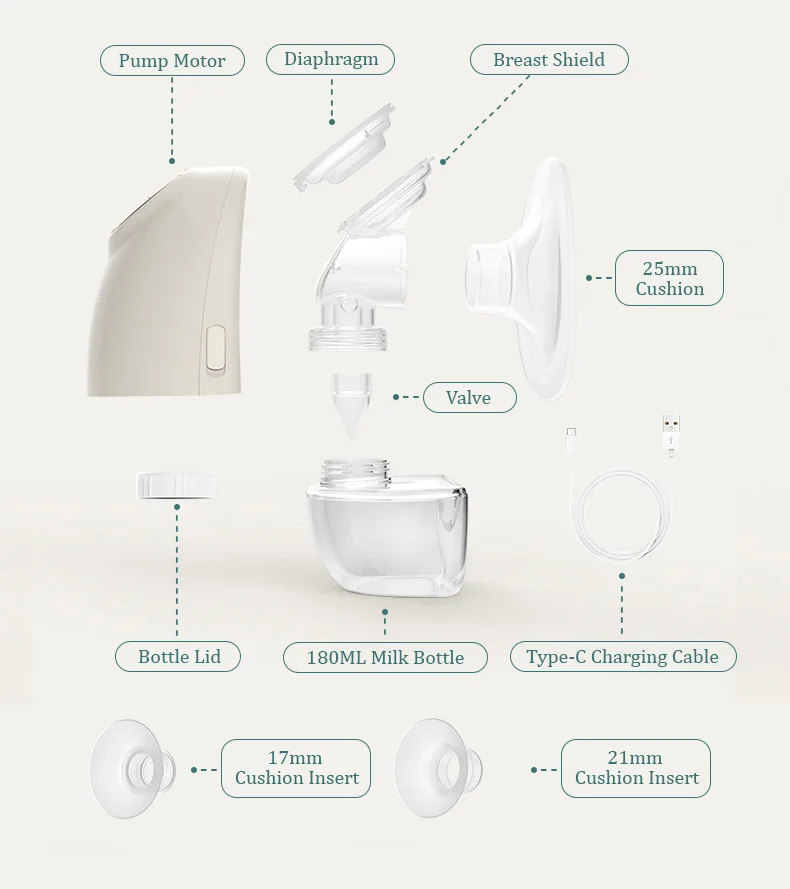**Detailed Description:**

The image features a meticulously arranged display of the various components of a breast pump, intended for expressing breast milk. Set against an off-white background, the parts are methodically spaced out from left to right, starting at the top.

- **Top Row (Left to Right):**
   - **Pump Motor:** An essential cream-colored device with a vertical switch, marked by an ovular label at the top featuring green text that reads "Pump Motor."
   - **Diaphragm:** This round white piece is to the right of the pump motor.
   - **Breast Shield Assembly:** Positioned under the diaphragm, consisting of a breast shield that connects to another round piece leading to a tube, which then connects to a threaded piece at the bottom.
   - **25mm Cushion:** Located to the right of the shield assembly, it resembles a satellite with a narrow left side that branches out to a wider, circular right side.

- **Center Section:**
   - **Threaded Valve:** Centrally placed, this component features threading at the top and tapers into a V-shape towards the bottom.

- **Bottom Row (Left to Right):**
   - **Bottle Lid:** A round white lid with ribbed sides for easy gripping.
   - **180ml Milk Bottle:** Right next to the lid, this small container has threading at the top and is marked with "180ml milk bottle."
   - **Charging Cable:** A Type-C charging cable, neatly wound into a circle, with both ends visible.
   - **Cushion Inserts:**
      - **First Cushion Insert:** Positioned below the bottle and cable, it is larger, round on the left, smaller, round, and threaded on the right. It is hollow.
      - **Second Cushion Insert:** To the right of the first insert, this 21mm cushion insert is nearly identical but slightly larger.

This detailed arrangement helps visualize each part clearly, ensuring an understanding of the breast pump's components and their relative positions.